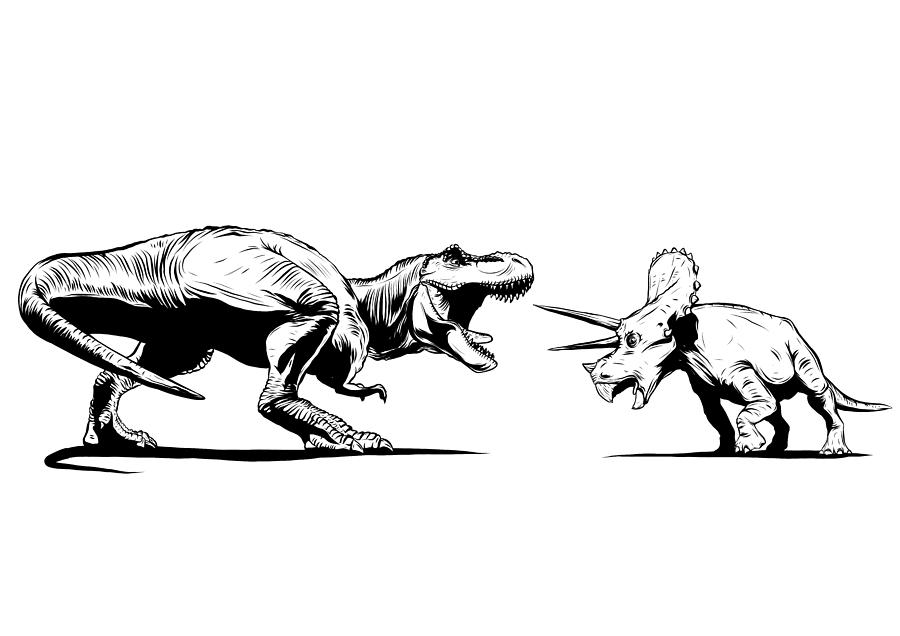In this black and white illustration, we observe a dramatic confrontation between two dinosaurs, rendered in a distinctive cartoon-animated style against a white background. Dominating the left side of the image is a formidable Tyrannosaurus rex, depicted in a threatening posture. This large dinosaur is crouched on its two powerful hind legs with its tail elevated and mouth wide open, exposing a series of sharp teeth and a visible tongue, suggesting a loud roar. Its tiny front limbs are curled and unable to touch the ground, adding to its menacing stance. The T-Rex’s upper body is white, while its underbelly is shaded black.

Opposing the T-Rex on the right is a much smaller dinosaur resembling a Triceratops. This diminutive yet defiant creature stands firmly on all four legs, displaying two prominent horns on its forehead. It has a short, skinny tail and a frilly neck, and its body structure is low to the ground, giving it a stout appearance reminiscent of a hippopotamus. Despite its size, the smaller dinosaur faces the T-Rex head-on, creating a tension-filled scene as if the two are about to engage in an imminent battle. The intricate details and contrasting sizes of the dinosaurs add a dynamic and intense atmosphere to the illustration.